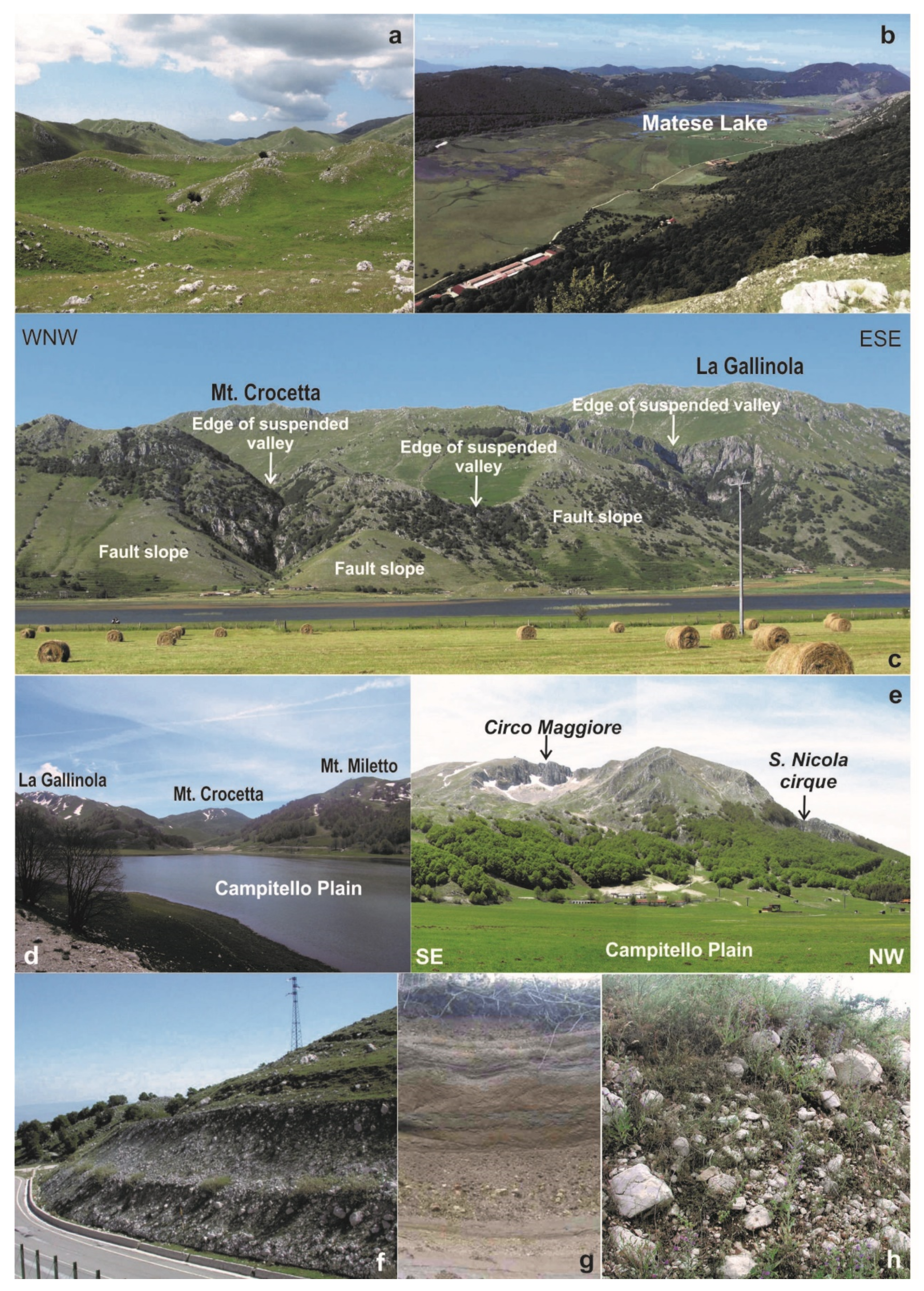This collage showcases a sequence of outdoor areas, labeled from A to H, capturing diverse landscapes and geological features. Each labeled section presents distinct natural vistas:

- **A**: A scenic view of mountains under an open sky, with the annotation indicating a fault slope, suggesting seismic activity.
- **B**: Matisse Lake, a partially dried lake exhibiting more green than blue hues, surrounded by plains and backed by mountains.
- **C**: The edge of a suspended valley near Mount Croqueta and La Gallinola, featuring flat areas with haystacks and a panoramic mountain backdrop.
- **D**: The Campitello Plain, showcasing another perspective of La Gallinola, Mount Croqueta, and Mount Mileto, with a stream flowing through the plain.
- **E**: The rugged terrain of Circo Maggiore and Nicola Cirque, a plain with mountains and a crater-like formation.
- **F**: A winding highway flanked by a tall mountain, indicating possible erosion areas with numerous rocks along the roadside.
- **G**: A close-up view of a dirt formation, revealing the texture and composition of the soil.
- **H**: A detailed shot of rocks interspersed with grass and leaves, highlighting the interaction between flora and the rocky surface.

This detailed description combines each element from the individual captions to create a cohesive and comprehensive portrayal of the diverse geographic and geological features represented in the collage.